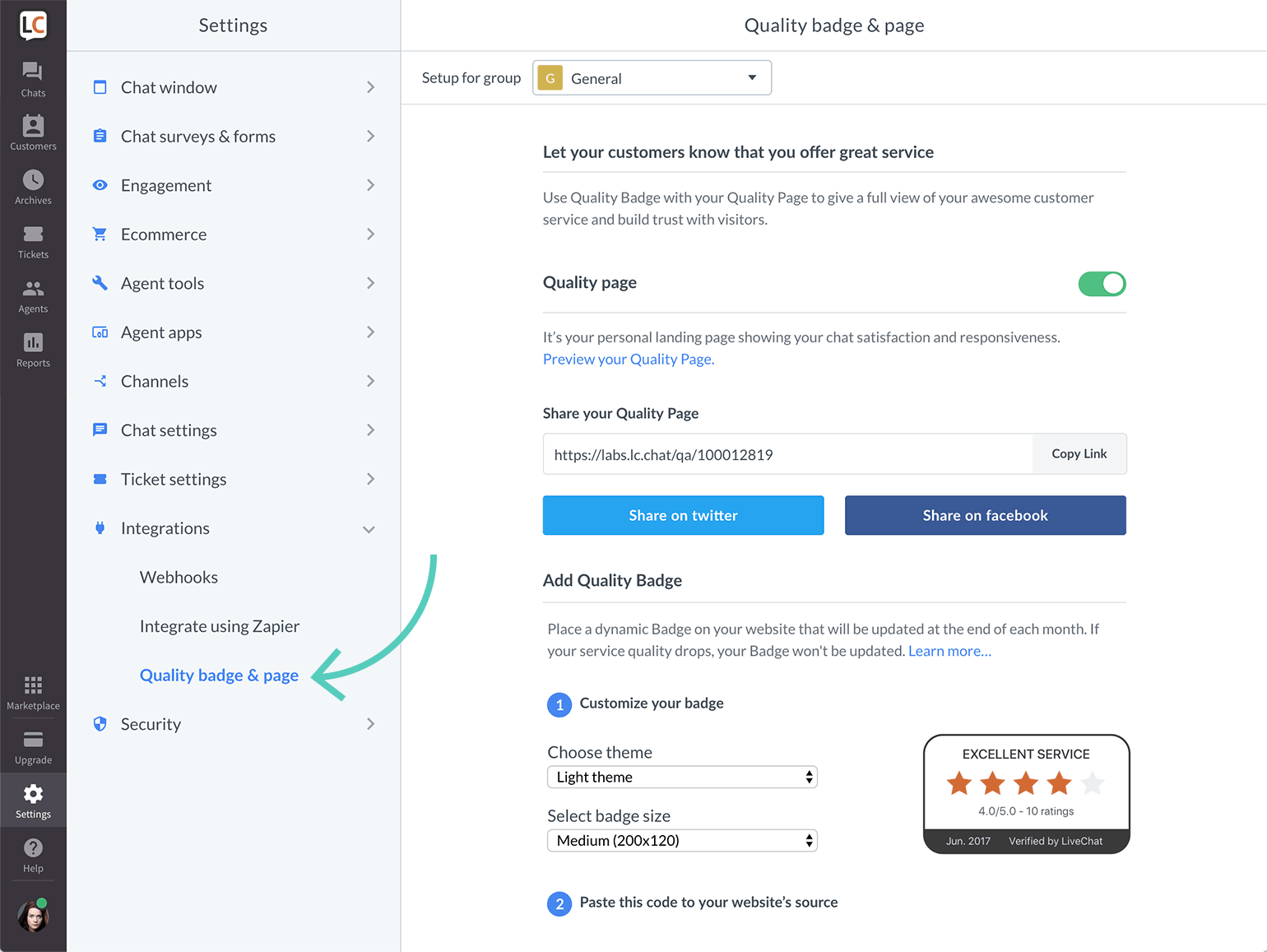The image depicts a complex user interface for a chat application's settings page, specifically focusing on "Quality Badges and Page."

On the left side of the screen, there's a menu with various settings options, each item accompanied by a right arrow. The list includes: 

- Chat Window 
- Chat Surveys and Forms
- Engagement
- E-commerce
- Agent Tools
- Agent Apps
- Channels
- Chat Settings
- Ticket Settings
- Integrations

The option "Integrations" has been expanded to reveal sub-options such as "Webhooks" and "Integrate Using Zapier."

Highlighted in blue within this menu is "Quality Badges and Page," indicating the user is currently navigating this section. A green arrow, clearly added via photo editing software, points to this highlighted option.

On the right side of the interface, the heading "Quality Badges and Page" confirms the current section. At the top, there's a header labeled "Set up for Group" with a dropdown menu in the "General" category.

The main content area reads: "Let your customers know that you offer great service. Use quality badges with your quality page to give a full review of your awesome customer service and build trust with visitors." Below this, there's a toggle switch labeled "Quality Page," which is currently turned on and displayed in green.

Further down, the text explains, "It's your personal landing page, show your chat satisfaction and responsiveness." There's a blue button below this labeled "Preview Your Quality Page."

At the bottom, the section "Share Your Quality Page" includes a data field with the URL "https://labs.lc.chat/qa/10012819," followed by a "Copy Link" button for easy sharing.